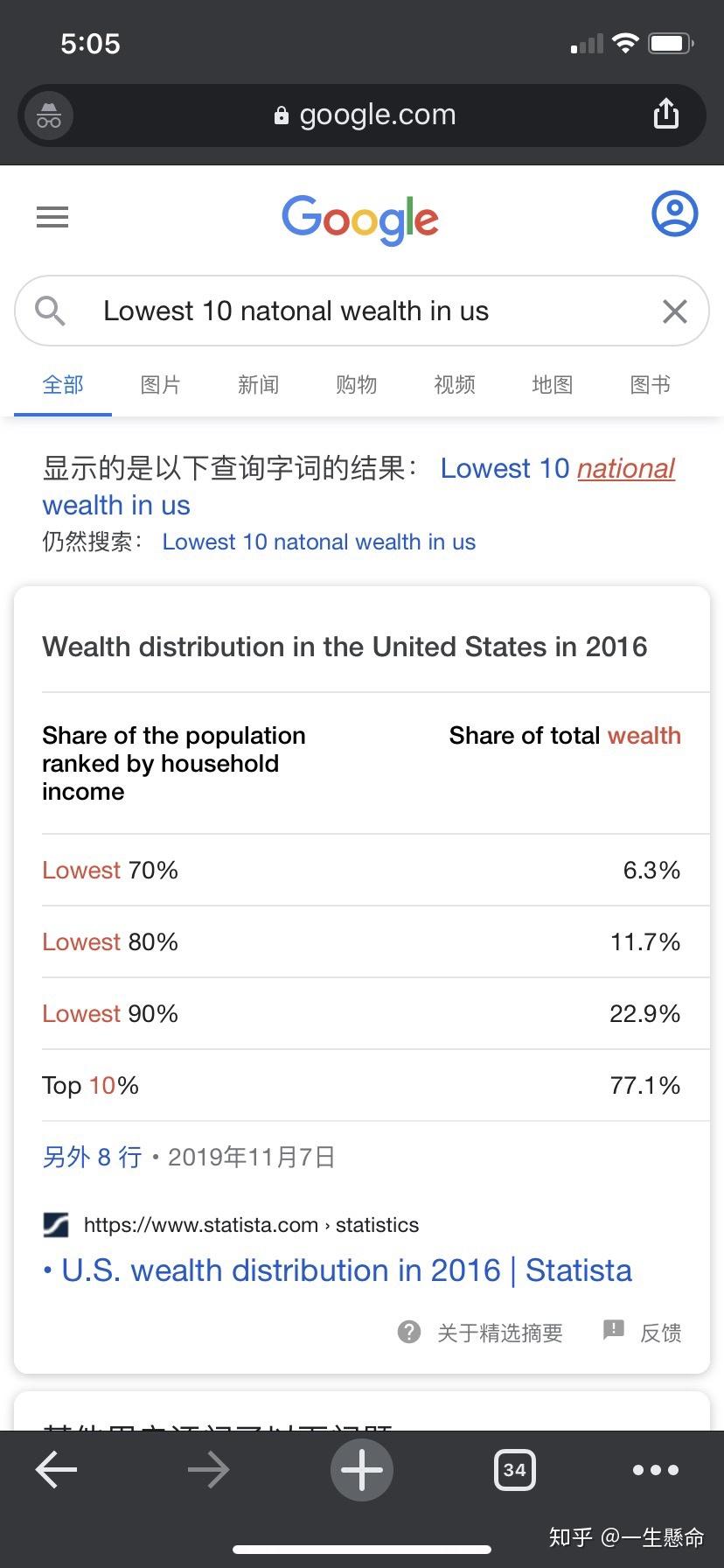This cell phone screenshot captures a Google search page. At the top center, the iconic Google logo is displayed with the letters "G" in blue, "O" in red, "O" in yellow, "G" in blue, "L" in green, and "E" in red. Just beneath the logo, the search bar contains the query "lowest 10 national wealth in the U.S." Below the search bar, the page transitions to content with various tabs written in what appears to be Chinese characters. 

Following this section, an English title in dark gray reads "Wealth distribution in the United States in 2016." This section is further divided into two main categories: on the left, "Share of the population ranked by household income," and on the right, "Share of total wealth," with the word "wealth" highlighted in red while the rest remains in gray. 

Additional breakdowns provide detailed percentages: 
- At the top of these categories, "Lowest 70%" is listed on the left side in gray, paired with "6.3%" on the right side.
- Below that, "Lowest 80%" appears on the left with "11.7%" on the right.
- Further down, "Lowest 90%" is positioned on the left, matched with "22.9%" on the right.
- At the bottom of the ranking, "Top 10%" is noted on the left, accompanied by a significantly higher "77.1%" on the right.

This visually organizes data regarding wealth distribution across different population segments in the United States for the year 2016.